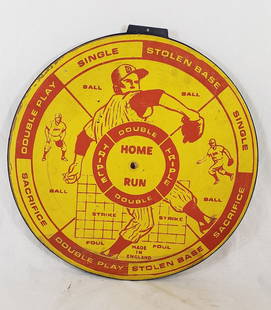This photograph showcases a vintage, circular game piece, primarily adorned in vibrant yellow with red fonts and details. Set against a white background, the piece appears to be a spinner with a central hole likely intended for a missing dial or spinner mechanism. Dominating the center of the piece is a dynamic illustration of a baseball pitcher in mid-throw, accompanied by the text "Home Run." The design is sectioned into four quadrants, each meticulously labeled with game-related terms: "Single, Stolen Base, Single, Sacrifice, Stolen Base, Double Play, Sacrifice, and Double Play." Surrounding the central illustration are additional labels indicating "Double" and "Triple." The piece, potentially part of a larger vintage game, is rich in sporting imagery and terminology, contributing to its nostalgic charm.